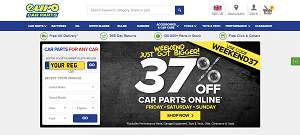This image is an enlarged, zoomed-out screenshot of a web page, viewed on a desktop, smartphone, laptop, or tablet. The left-hand side of the image features white text spelling "e u i r o" in lowercase letters. Beneath this text, a blue rectangle is partially visible, although it is blurred and somewhat indecipherable; it appears to contain elements related to "car," "yellow," and some inner parts.

On the right-hand side, a search bar is prominently positioned, accompanied by a square icon bearing a white magnifying glass. At the top, several blurred menus in white text are present, but the distance and quality of the screenshot make the text illegible. Adjacent to the search bar, the top right section includes a small UK flag with a blue background and red crisscross lines.

Further to the right, there's a pin icon, a silhouette icon likely representing a login option, and a basket icon which seems to be a shopping cart. This basket icon is tagged with a yellow label, presumably displaying the number of items in the cart.

The central portion of the webpage showcases a white rectangle set within a larger black rectangle. Inside the white rectangle, the text "CAR PARTS" appears in bold blue, while "FOR ANY CAR" is bolded in red, both sections in all uppercase letters. Below this, a black rectangle contains text that is too blurry to read, even when zoomed in.

A blue-to-yellow gradient rectangle includes the phrase "YOUR REG," accompanied by a square button with "GO" in white text. Below this, "or" is written in gray, followed by an invitation to fill out specific information.

In the main black area of the webpage, bold yellow text declares, "Weekend just got bigger," with the word "bigger" underlined for emphasis. Next to this, a sideways yellow rectangle with black text reads, "USE CODE" followed by bolder black text, "WEEKEND37."

Centralized in the black area, the text "37% OFF CAR PARTS ONLINE" is prominently displayed in bold white, with the percentage symbol creatively formed by two hubcaps and a wrench. Below, the text "Friday or Saturday or Sunday" is visible in yellow, and a yellow button with black text commands viewers to "SHOP NOW."